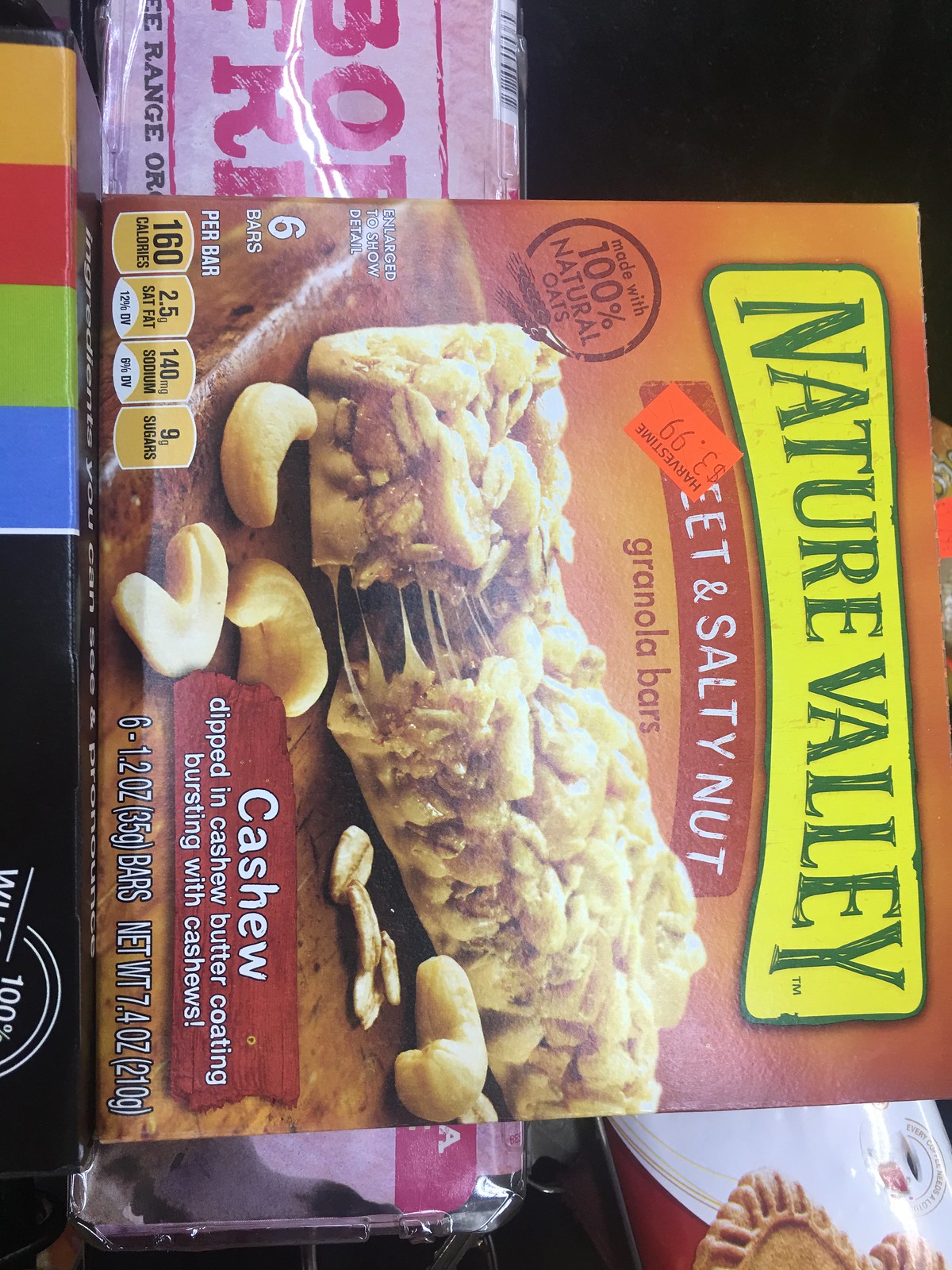The image prominently features a box of Nature Valley Sweet and Salty Nut Granola Bars. The center of the box displays the product name, surrounded by multiple informative labels and graphics. A price sticker on the box reads $3.99. On the left side, there's a circular logo stating "Made with 100% Natural Oats," with a reflective light effect. Below, another section of the box highlights the nutritional information: 160 calories, 2.5 grams of saturated fat, 140 milligrams of sodium, and 9 grams of sugars per bar. The box contains 6 bars, each weighing 1.2 ounces, for a total net weight of 7.4 ounces (210 grams).

To the right side of the box, text in brown lettering describes the flavor: "Cashew dipped in cashew butter coating, bursting with cashews." This is accompanied by an enticing image of one of the bars, showcasing its juicy and sticky texture, topped with various nuts and a layer of what appears to be caramel or cashew butter.

In the background, a pink rectangle contains additional text, though the specifics are unclear. To the left of this, another box is visible, featuring a vibrant mix of colors including yellow, red, green, and blue.